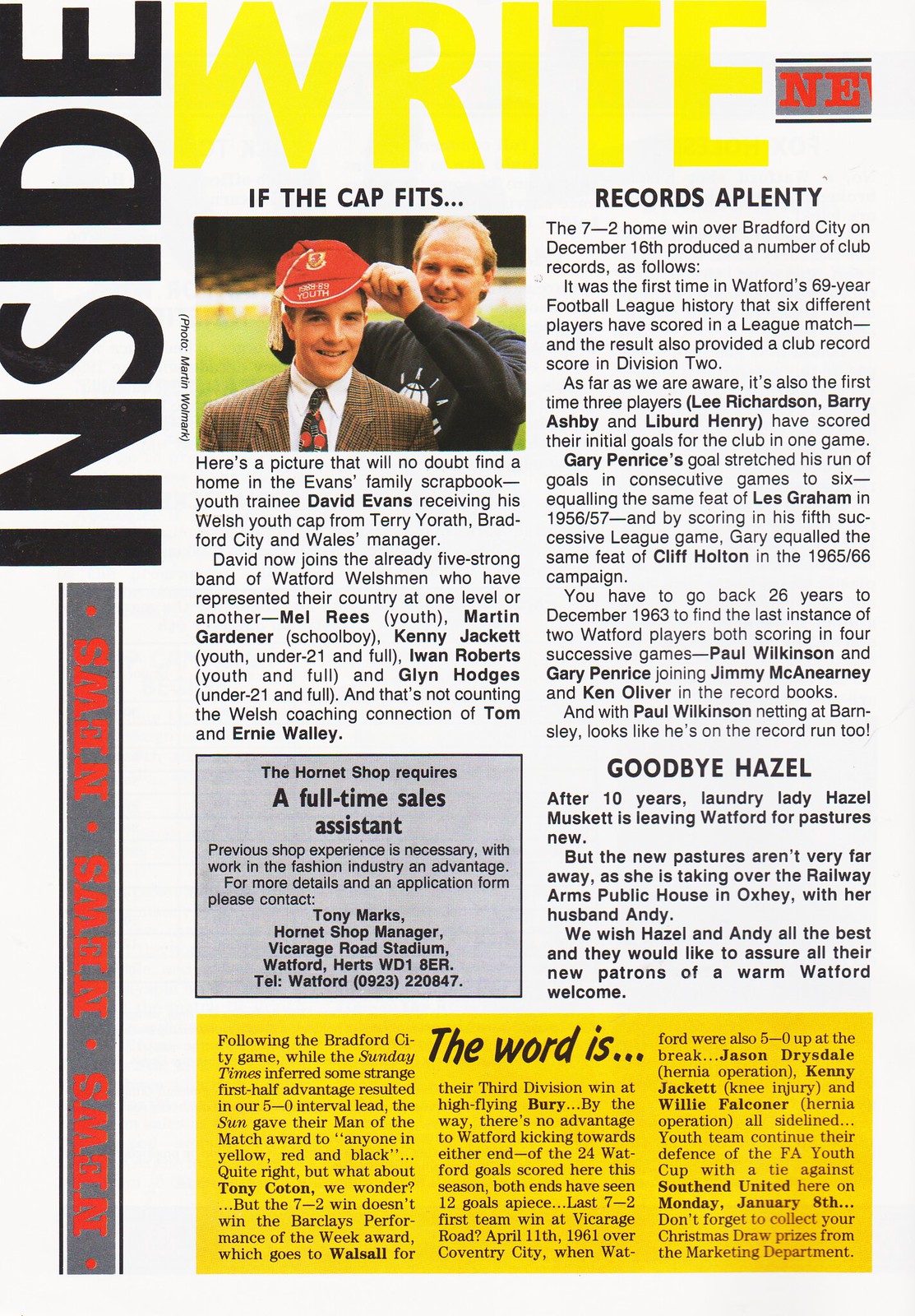The image appears to be the front cover of a sports magazine or newsletter with a white background. The word "INSIDE" is displayed vertically in black lettering along the left-hand side, and the word "RIGHT" is prominently featured in yellow at the top. There are two main columns of stories; the left column's top headline reads "If the Cap Fits" and features a heartwarming photo of a man placing a red cap on a boy. The caption details youth trainee David Evans receiving his Welsh youth cap from Terry Yorath, Bradford City and Wales manager, with the remark that this image will find a place in the Evans family scrapbook. Other mentioned individuals note that David has joined Watford's Welsh representatives. 

The right column includes another headline about "Records Aplenty," likely discussing various soccer records. Additionally, there's an ad for the Hornet Shop and a brief column at the bottom bidding farewell to Hazel Musket. The colors predominantly seen are white, black, gray, red, yellow, green, and tan, contributing to the sports-themed aesthetic.